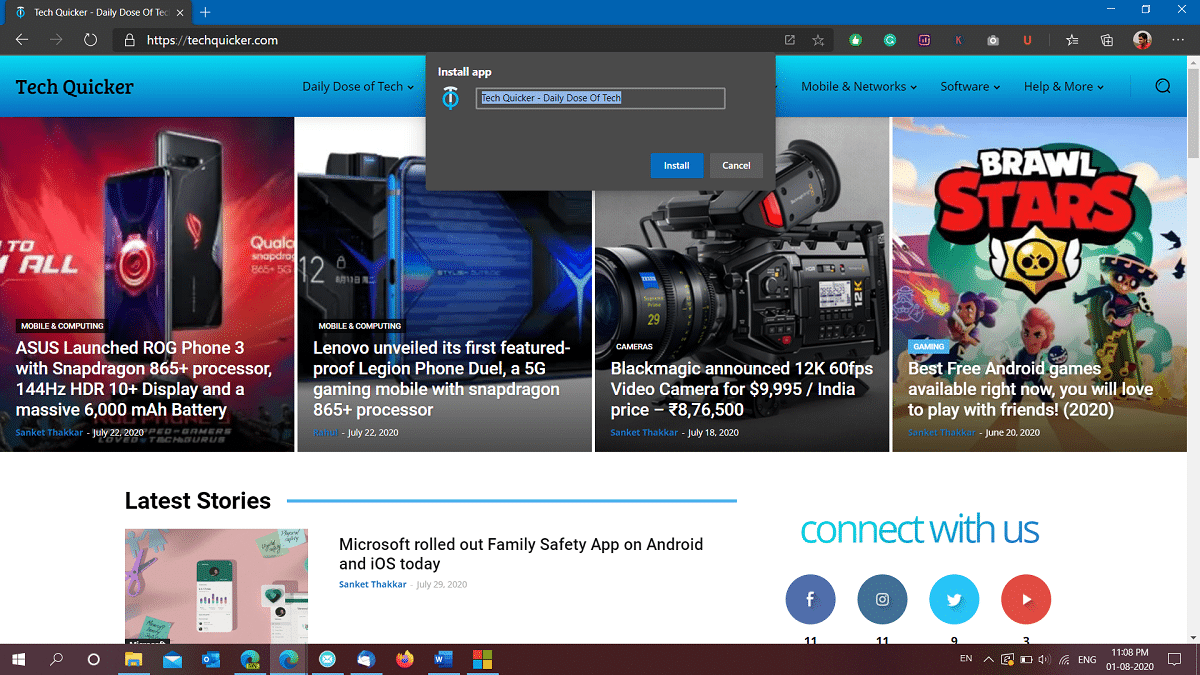This screenshot captures a section of the TechQuicker website. A black notification bar appears at the top, prompting users to install the app. The bar partially covers some of the site's illustrations as the installation process begins. Below the TechQuicker banner, there are four highlighted articles: ASUS's launch of the ROG Phone 3, Lenovo unveiling its first future-proof Legion phone, Blackmagic's announcement of a 12K 60fps video camera, and a feature on Brawl Stars as one of the best free Android games to play with friends in 2020. Further down, the site showcases its latest stories, including Microsoft's rollout of the Family Safety app for both Android and iOS phones. Navigation options to explore different sections of the website are available at the top.